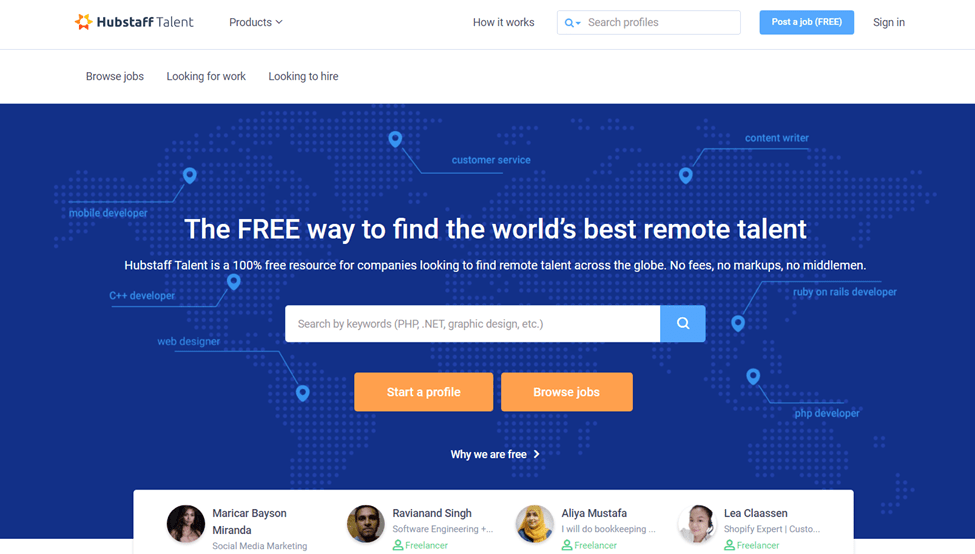The image depicts a webpage from Hub Staff Talent, featuring an orange sun icon in the top left corner. To its right are navigational elements, including a "Products" tab with a downward arrow, followed by a "How It Works" link, and a search bar labeled "Search Profiles." A blue button marked "Post a Job (Free)" and a "Sign In" option are also visible. Below this navigation bar, a white section presents options like "Browse Jobs," "Looking for Jobs," and "Looking to Hire."

Further down, the design transitions to a blue background resembling a world map illustrated with tiny blue dots representing countries. Overlaid text promotes Hub Staff Talent as "The Free Way to Find the World's Best Remote Talent," emphasizing that the service is "100% free" with "No fees, no markups, no middlemen." 

Various job titles such as Mobile Developer, C++ Developer, Web Designer, Customer Service, Content Writer, Ruby on Rails Developer, and PHP Developer are scattered across the map with directional arrows. Additionally, the page contains a search bar and several orange buttons. Lower on the page, there are profile examples featuring individuals' photos, names, and job positions.